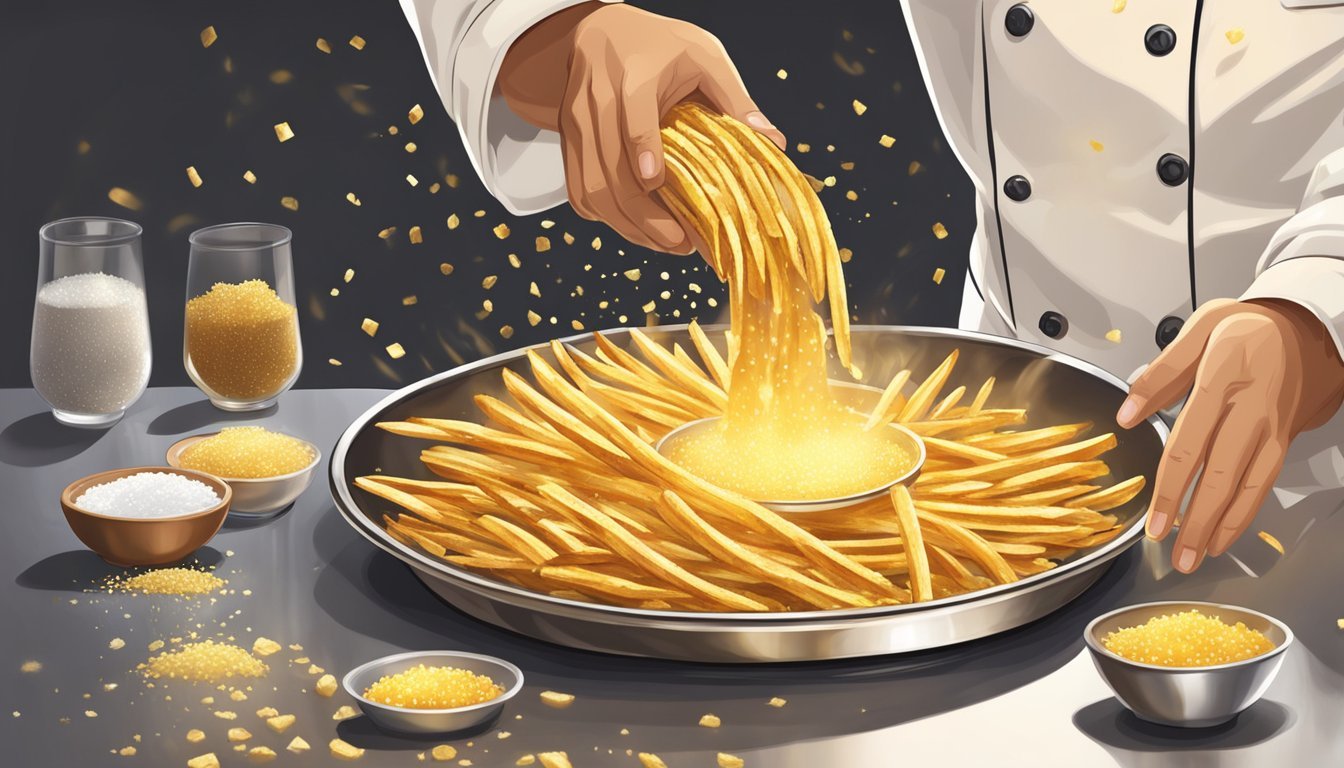The image is a detailed drawing of a chef, depicted from the shoulders down, wearing a white chef's jacket with two rows of black-trimmed buttons; six buttons on the front are visible. The chef's right hand, visible from the upper left center, is holding French fry-shaped items that appear to be potato strips, and he is pouring them into a large bowl filled with a yellow liquid, likely hot cheese, in the center of the image. His left hand, seen from the upper right corner, helps guide the fries into the bowl. Other French fry-shaped items are already in the large bowl, being coated in the yellow liquid. Two glasses reside in the upper left portion of the picture, one containing a white granular substance, the other holding a gold-colored grain. Below these glasses are two small bowls, one white and one brown, containing similar granular substances. Additionally, two smaller silver bowls containing the same granular substances are positioned in the left and right corners of the image. The setting includes a silver tray and smaller cups filled with various kinds of cheese. The table is sprinkled with bits of cheese, complementing the culinary theme of the artwork.